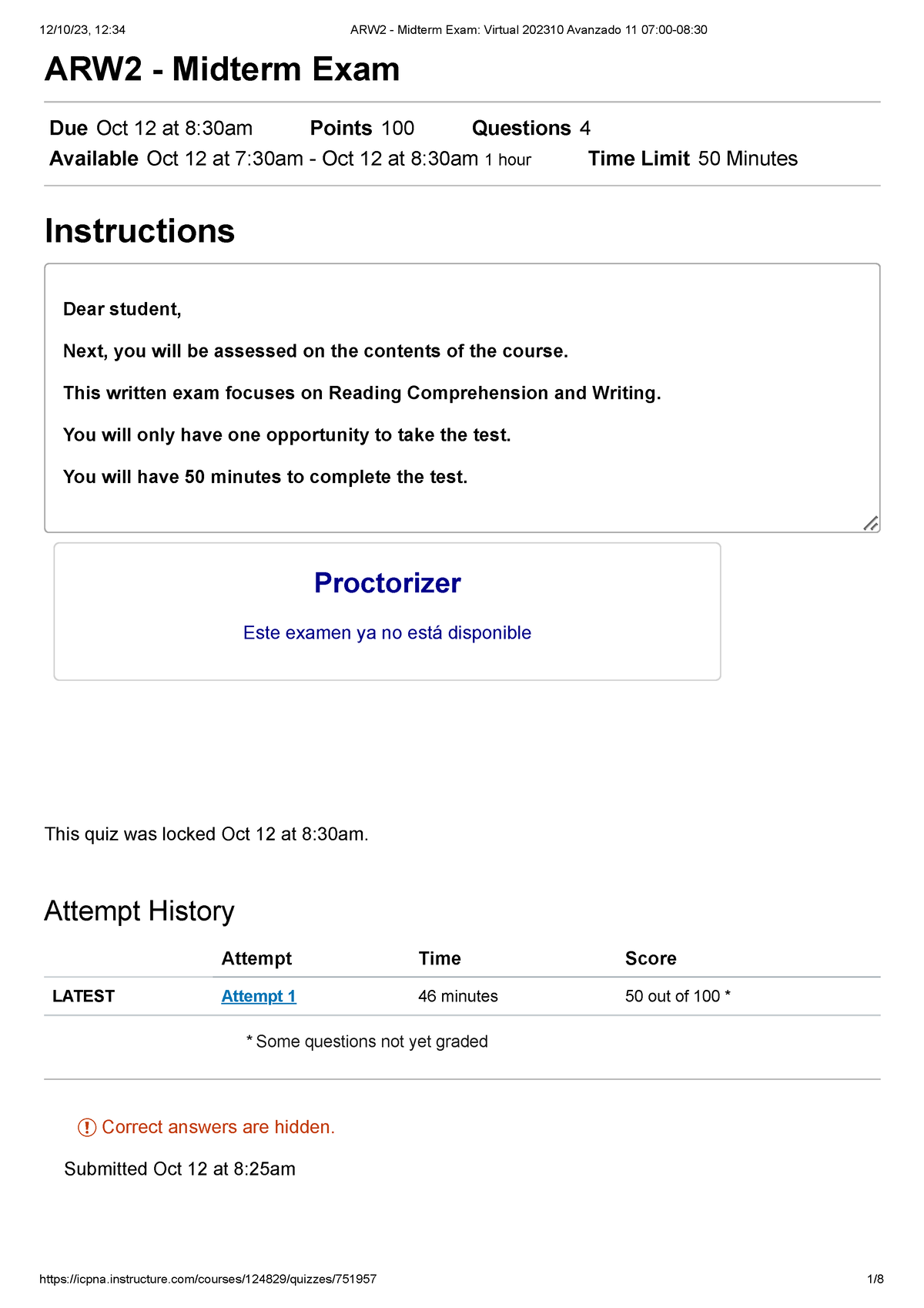This is an image of a midterm exam screen capture displayed on a white background with black lettering. The header indicates "ARW II Midterm Exam, Virtual 2023," scheduled for December 10, 2023, from 7:00 AM to 8:30 AM. The exam is due on October 12th at 8:30 AM, with a total of 100 points distributed over four questions. The exam window is open from October 12th at 7:30 AM to October 12th at 8:30 AM, providing a one-hour time limit of 50 minutes for completion.

Instructions follow: "Dear Student, you will be assessed on the course contents. This written exam focuses on reading comprehension and writing. You have only one opportunity to take the test and 50 minutes to complete it."

In blue text, it states, "Proctorizer este examen ya no está disponible" (indicating the exam is no longer available, likely in Spanish). Below this, it notes: "This quiz was locked on October 12th at 8:30 AM."

Further down, under "Attempt History," the latest attempt shows a blue hyperlink labeled "Attempt 1." The details for this attempt include a duration of 46 minutes and a score of 50 out of 100, with an asterisk denoting that some questions are not yet graded.

In orange or red text, a message reads: "Correct answers are hidden!" with an exclamation point. The submission timestamp is noted as October 12th at 8:25 AM.